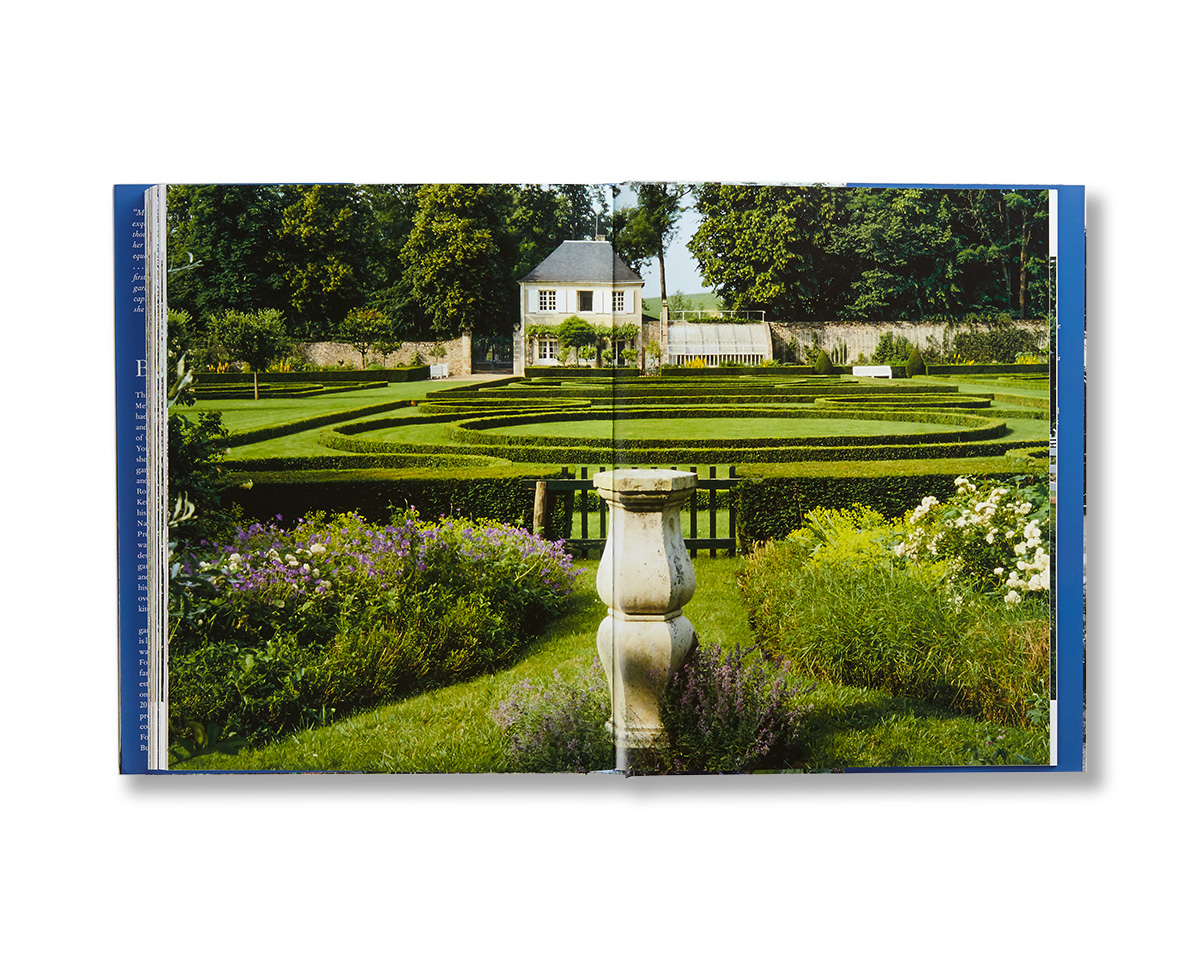This image displays an open booklet with both pages depicting a detailed illustration of an English estate and its garden, set against a white background. The central focus is a two-story cottage with white shutters and a gray roof. The front of the house is adorned with green vines climbing up its facade. To the right of the house, a greenhouse is visible, surrounded by lush grass, trees, and a carefully landscaped garden. The garden features an intricate maze-like layout formed by low-lying, neatly trimmed hedges and small shrubs. In the bottom right, green shrubs with white flowers are prominent, complemented by violet flowers scattered throughout the scene. There is also a stone pedestal in the foreground, flanked by two plants with violet blooms. A gate and a sculpture add further detail to the walk-through garden space, with a clear walkway leading up to the gate, and the scene is illuminated by daylight, suggesting a late evening ambiance.